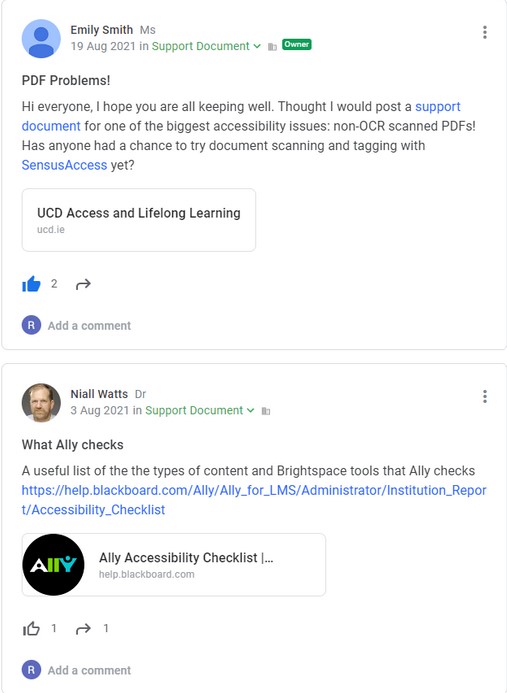This screenshot captures a conversation thread discussing issues with PDF accessibility. The vertical screenshot consists of two primary sections: one is a support documentation post by Ms. Emily Smith dated August 19, 2021, and the other is a post by Dr. Niall Watts.

In the first section, Ms. Smith, addressing the community with a friendly greeting, introduces the support document titled "PDF Problems." The document mentions a significant accessibility issue with non-OCR scanned PDFs and provides a clickable link for further details. She also inquires if anyone has tried using Census Access, which is also linked for easy access. The post is highlighted with a rectangular box stating "UCD Access and Lifelong Learning," indicating it as another clickable link. The post has received two thumbs up, and options are available to forward or comment on it.

Directly below, Dr. Niall Watts's post, titled "What Ally Checks," provides a useful list of all types of content and tools in Brightspace that Ally examines. It includes a clickable link to an institution report and an accessibility checklist hosted on help.blackboard.com. This post has garnered one thumbs up with options for forwarding.

The conversation thread is visually structured with interactive elements and helpful resources aimed at improving document accessibility.